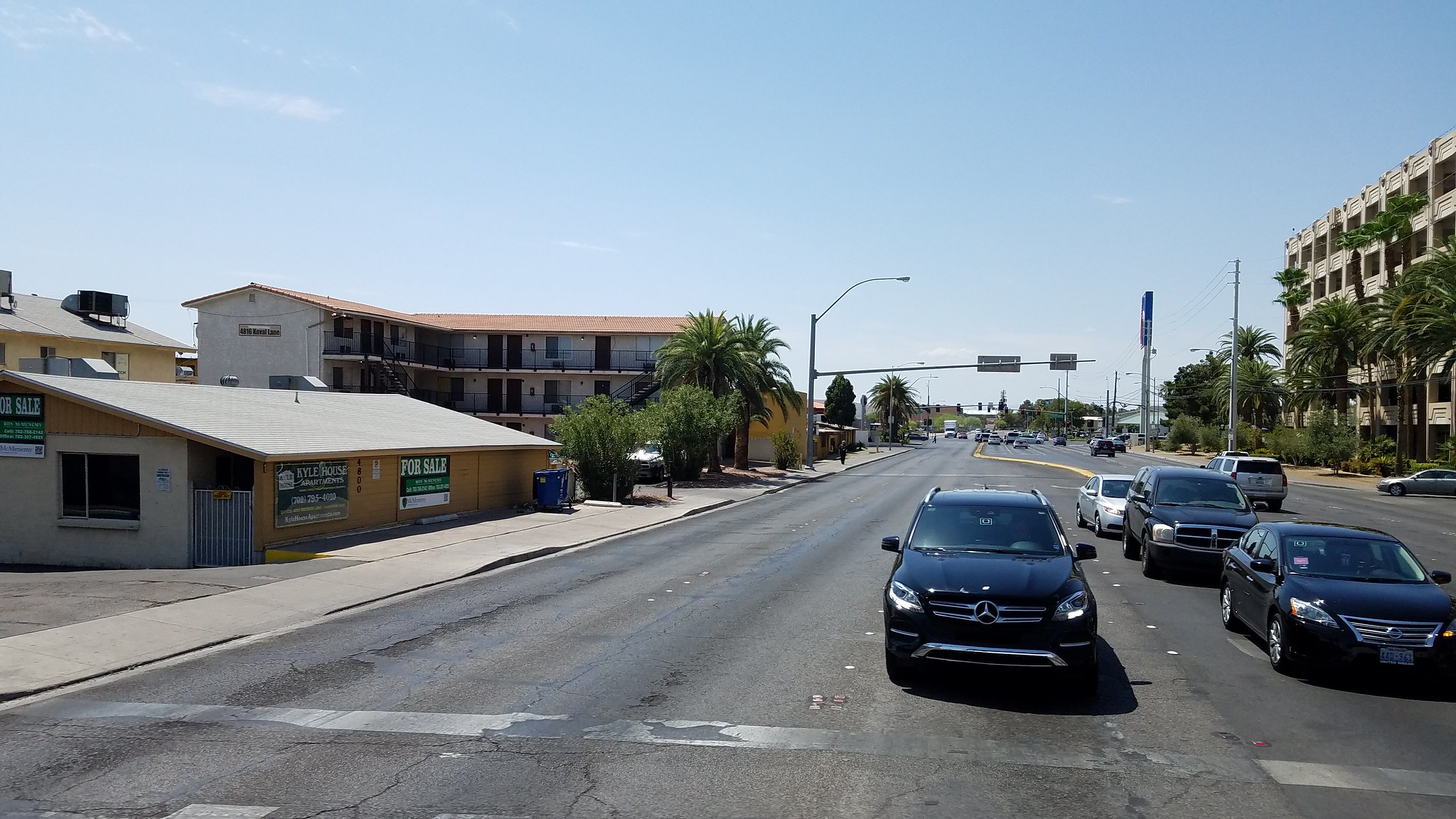The photograph captures a bustling intersection with several cars stopped, forming an orderly line. The image has a rectangular format, with the longer sides running horizontally. At the top of the image, a light blue sky dotted with small white clouds creates a serene backdrop. 

Dominating the right side of the frame is a large, five-story building that serves as an outdoor parking garage. The structure is made of tannish concrete, featuring numerous window openings without glass, allowing a view into its interior. In front of the garage stands a row of lush green palm trees, adding a touch of nature to the urban scene.

The center of the photograph showcases a multi-lane road with gray asphalt, segmented by small metal or plastic dividers. Towards the bottom of the image, a long white stop line—now faded with black spots and missing sections—indicates where vehicles need to halt. Positioned at the intersection, five cars are lined up, waiting for the traffic light (which is out of the frame) to change.

This detailed depiction of an urban intersection balances architectural elements with natural components, capturing a typical moment in city life.